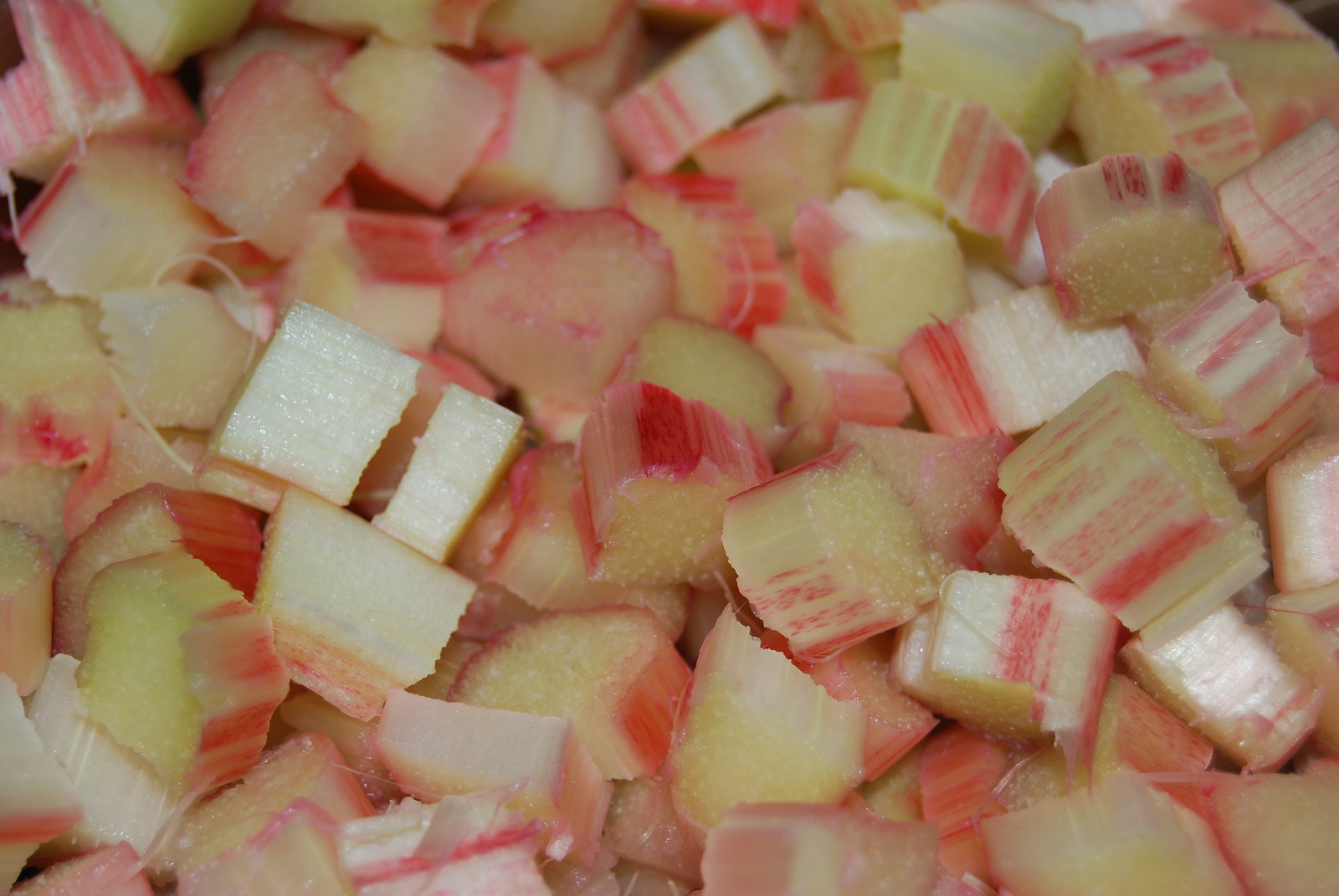The image is a close-up photograph of small, diced rhubarb pieces scattered across the entire frame. The rhubarb chunks, each approximately the size of a dime and about half an inch thick, display a variety of colors from light red to yellowish-green. The outer edges show a thin red skin, while the interiors reveal a pale green to yellowish flesh. The pieces are moist and reflective, indicating their freshness. Fine fibrous strands are visible where the pieces have been cut. The lack of perspective and the uniformity of the diced portions make it challenging to determine the exact size, but they appear small, suggesting the rhubarb may have been harvested before fully maturing. The image captures the vibrant texture and intricate details of the rhubarb, emphasizing the contrasting colors and fresh appearance of the vegetable.